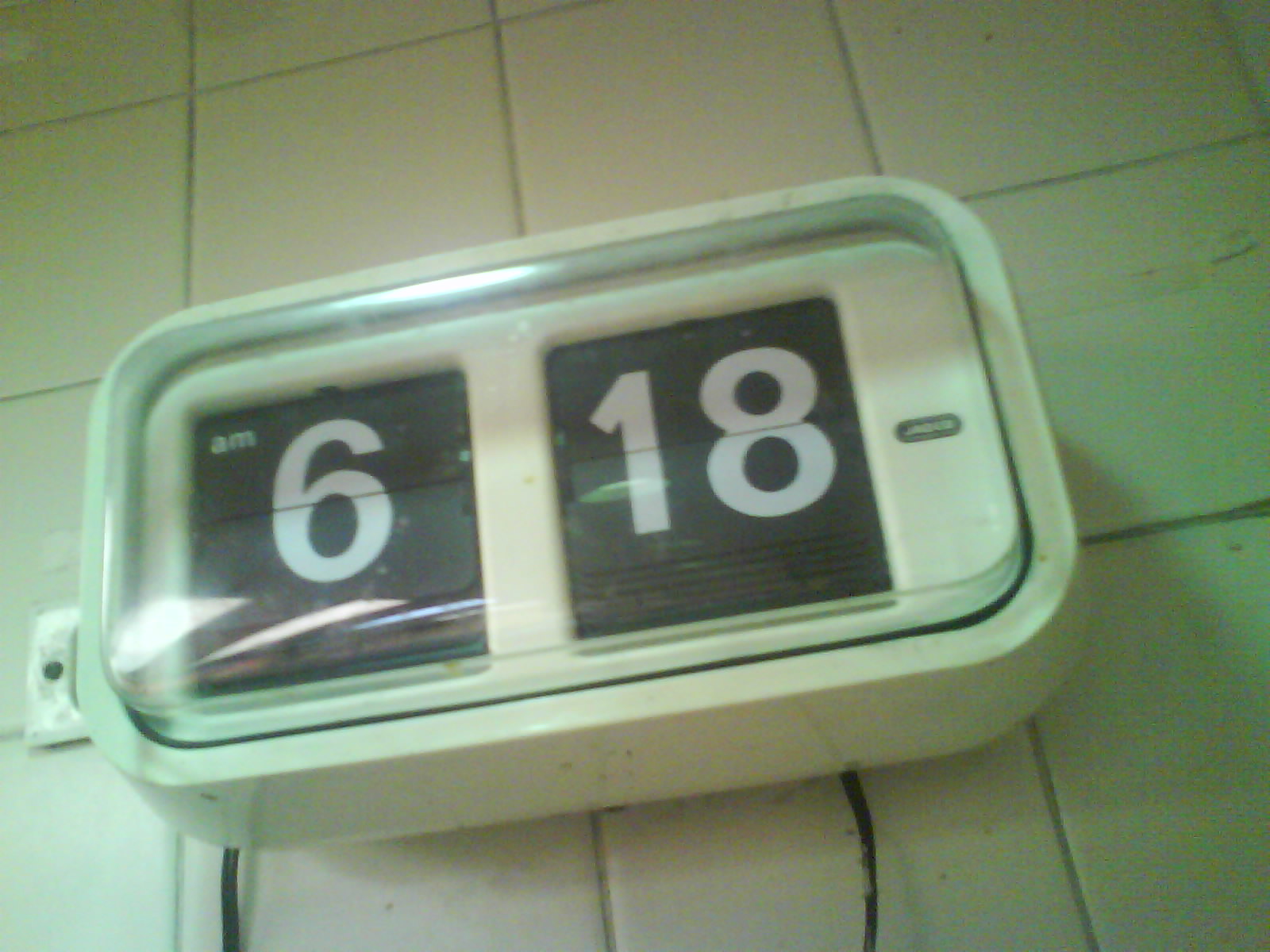The image depicts a large, bulky rectangular clock mounted on a wall composed of white or off-white tiles with visible grout lines and some missing sections. The clock features a clear transparent cover that reflects light, indicating illumination from behind the camera. Inside the clock, a Rolodex mechanism displays the time as 6:18 AM. The numbers are shown in white font on a black square background, with a small "AM" in the top left corner. The clock's design includes white plastic surrounding the numbers, further emphasizing its segmented display. Additionally, there are a couple of black wires hanging down from the clock. One tile in the background appears cracked, adding a touch of imperfection to the setting.